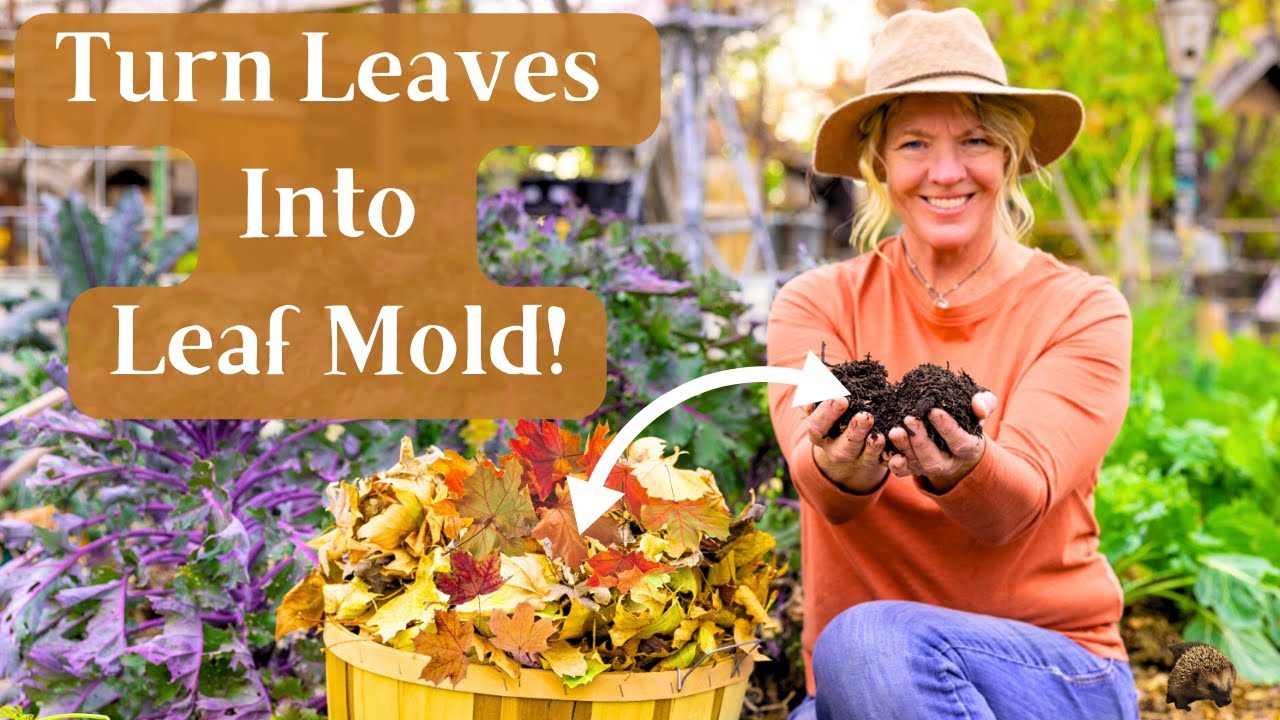In this gardening-themed image, a woman is kneeling on the ground, actively engaged in creating leaf mold. She is dressed in an orange long-sleeved shirt, blue jeans, and a brown wide-brimmed hat. Additionally, she sports a necklace and has blonde hair cascading under her hat. The woman is carefully holding a handful of mulch, demonstrating her gardening process. Beside her, a yellow basket brimming with vibrant yellow and red leaves signifies the raw materials for the leaf mold. 

The visual layout features instructional text on the left side, displayed against a brown background in white letters with the energetic exclamation, "Turn leaves into leaf mold!" White arrows graphically illustrate the transformation process, pointing from the mulch in the woman's hands to the leaves in the basket and vice versa.

Surrounding the scene, there is varied vegetation that enhances the lush backdrop. To the right of the woman, green foliage adds to the verdant charm, while to her left, a hint of purple plants introduces a pop of contrasting color. This detailed composition not only highlights the gardening activity but also situates it within a beautifully eclectic garden setting.